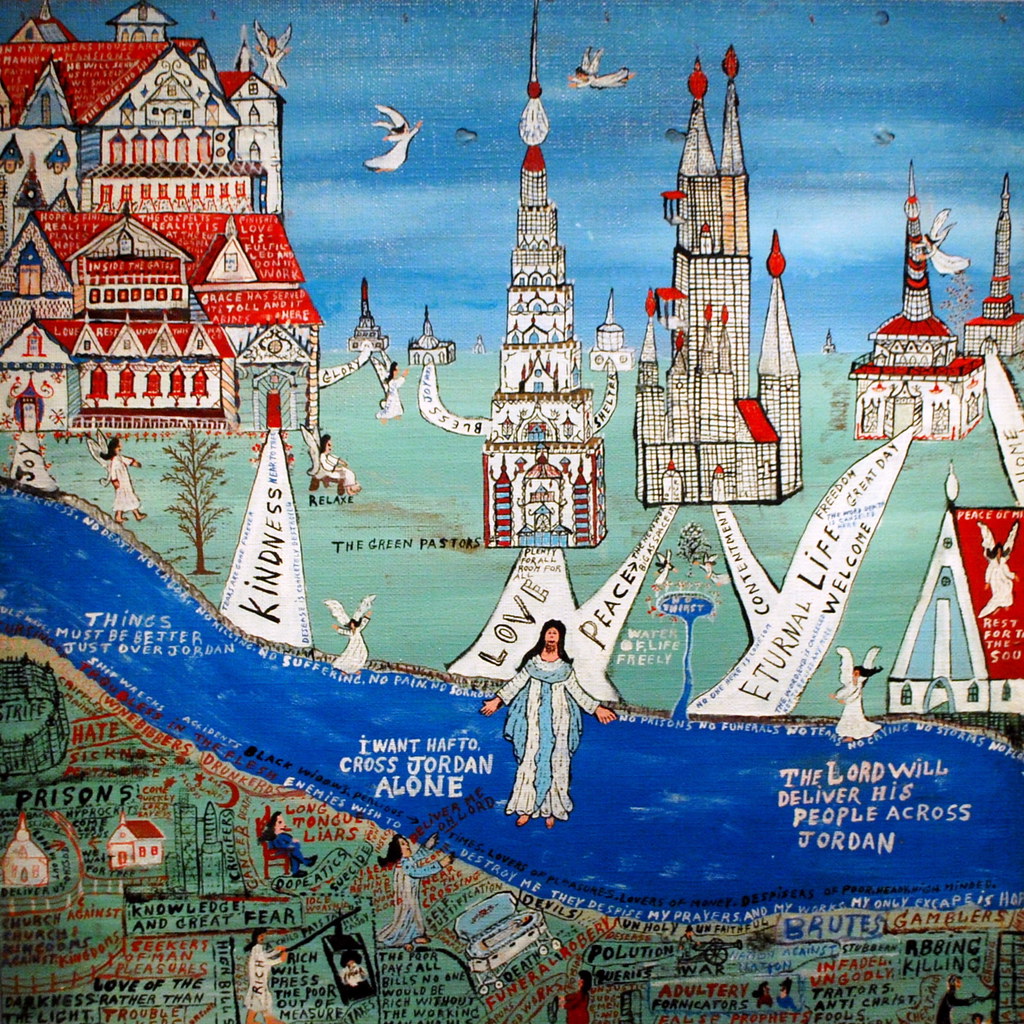The image is a detailed hand-drawn painting featuring a prominent blue river flowing from left to right, which appears to be rendered with dark blue ink and a purple marker. In the center of the scene, the river contains white text that reads: "Things must be better just over Jordan. I won't have to cross Jordan alone. The Lord will deliver his people across Jordan." 

In the middle of the river stands a figure, presumably Jesus, depicted with outstretched arms, wearing a blue and red outfit which some interpretations describe as a white gown with blue trappings. The background is a mix of a lush green field dotted with buildings resembling churches or castles with red roofs, all of which seem to symbolize places of worship or attainments of faith. 

The expansive blue sky is adorned with both black dots and angelic figures, some white and winged, signifying a heavenly presence. Around the green field, various paths are labeled with words like 'kindness,' 'love,' 'peace,' and 'eternal life,' suggesting conduits to higher virtues or spiritual goals. 

At the very bottom of the image against the green background, there are numerous textual elements that resemble graffiti and might contain Bible quotes or religious sayings, although some words appear misspelled or cut off. Among these elements, a person labeled "rich" stands towards the left, facing right with hands extended in front of him, symbolizing perhaps the separation between material wealth and spiritual salvation. 

Overall, the river seems to demarcate a divide between an earthly realm filled with sinners and paths leading to the metaphorical Kingdom of Heaven.